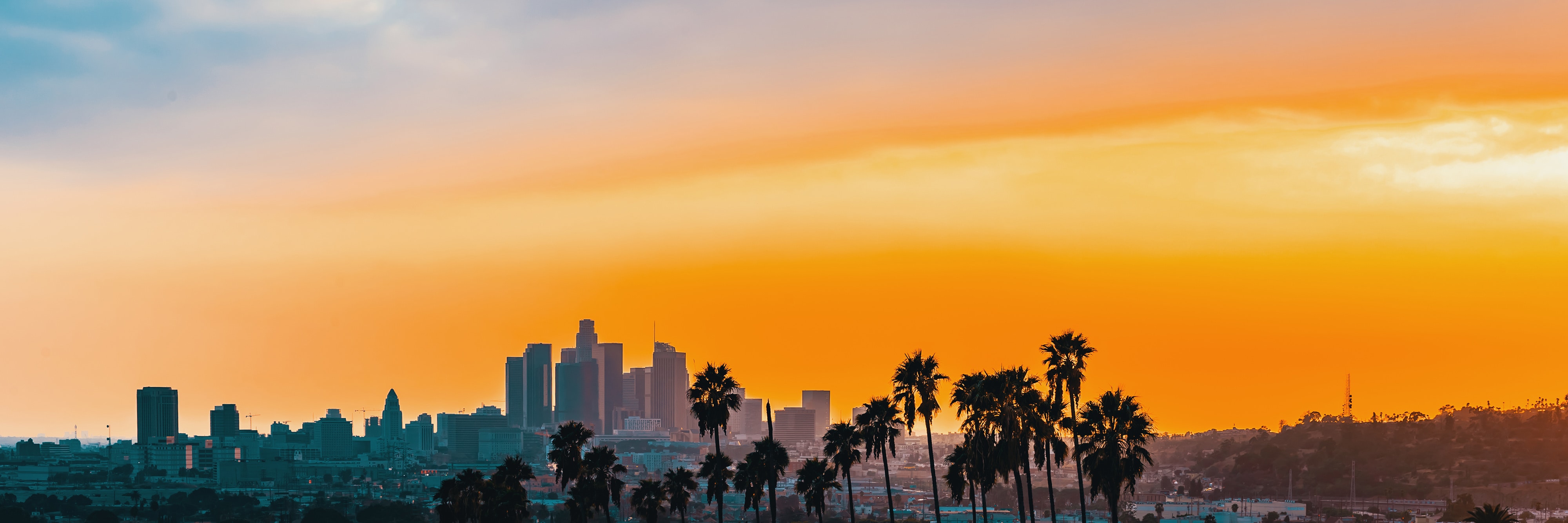A detailed aerial view showcases a sprawling downtown cityscape that appears to be either in Florida or California, possibly Los Angeles. The rectangular, horizontal composition reveals an abundance of tall buildings clustered centrally, tapering into smaller structures towards the left and expansive land with hilly terrain to the right. Dominating the foreground are numerous palm trees, approximately two dozen, creating a lush barrier before the urban sprawl. The sky is a striking blend of colors, transitioning from deep blue at the top to rich hues of orange and yellow, indicative of a setting or rising sun. This merging spectrum illuminates the city, with a noticeable reflection of sunlight on some high-rise facades. The left upper corner of the image features a prominent white sun, adding a layer of ethereal beauty to the scene. There’s a complexity and vibrancy to the image that requires close inspection to fully appreciate its depth and detail, revealing more with every zoom.